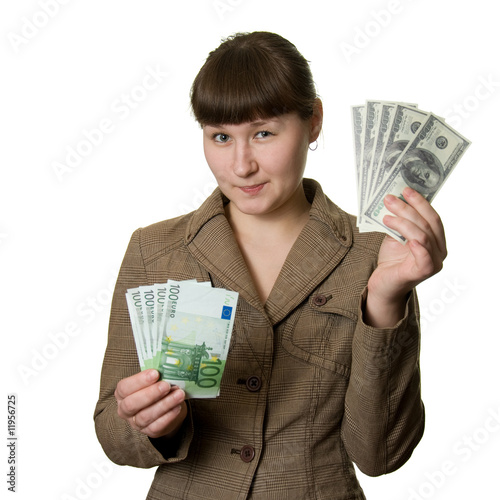In this image, a woman stands against a plain white background, marked with a faint, diagonal watermark reading "Adobe stock." She has short brown hair with long straight bangs, brown eyes, and a smirk on her face. She's wearing a light brown corduroy-style button-up coat. In her left hand, raised slightly higher, she holds five $100 American bills, fanned out. In her right hand, she holds several 100 Euro notes, their distinctive light and dark green colors visible, each bearing the image of what looks like the Arc de Triomphe. In the lower left-hand corner of the image, there is a vertical text that reads "Adobe stock" followed by the image number 11956725.